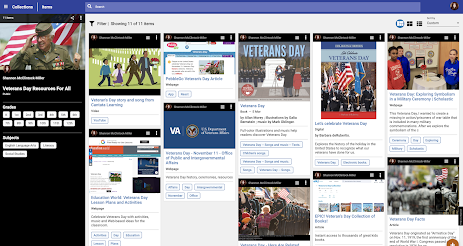This webpage features a rectangular layout with a white background. On the top left, there is a black vertical rectangle adjacent to the white section, giving the appearance of a merged design. Dominating the upper section is an image of a soldier holding an American flag behind his back while saluting, symbolizing respect and honor.

Across the page, a sequence of photos commemorates Veterans Day. These visuals are interspersed with brief written paragraphs in black and blue font, though the text is too small to read clearly. In the center, bold light blue letters prominently spell out "Veterans Day," emphasizing the webpage's focus.

The first photo in the series shows a family—a husband and wife with two children—strolling across a field. The daughter is dressed in a blue dress and white jacket, while the son wears blue and black pants with a blue shirt or jacket. The following image contains only text, followed by the central Veterans Day photo.

Next in line is a picture of soldiers standing beside American flags. Another image depicts a classroom setting with a table in the foreground. In this scene, a little boy in a red shirt and another in a blue shirt are seen on the left, while an adult, possibly a teacher or parent in a blue shirt, is on the right.

Below these images, most of the content consists of text. The third image in this lower section features a group of people, while the final image showcases a black-and-white composition with an American flag, tying back to the theme of national pride and remembrance.